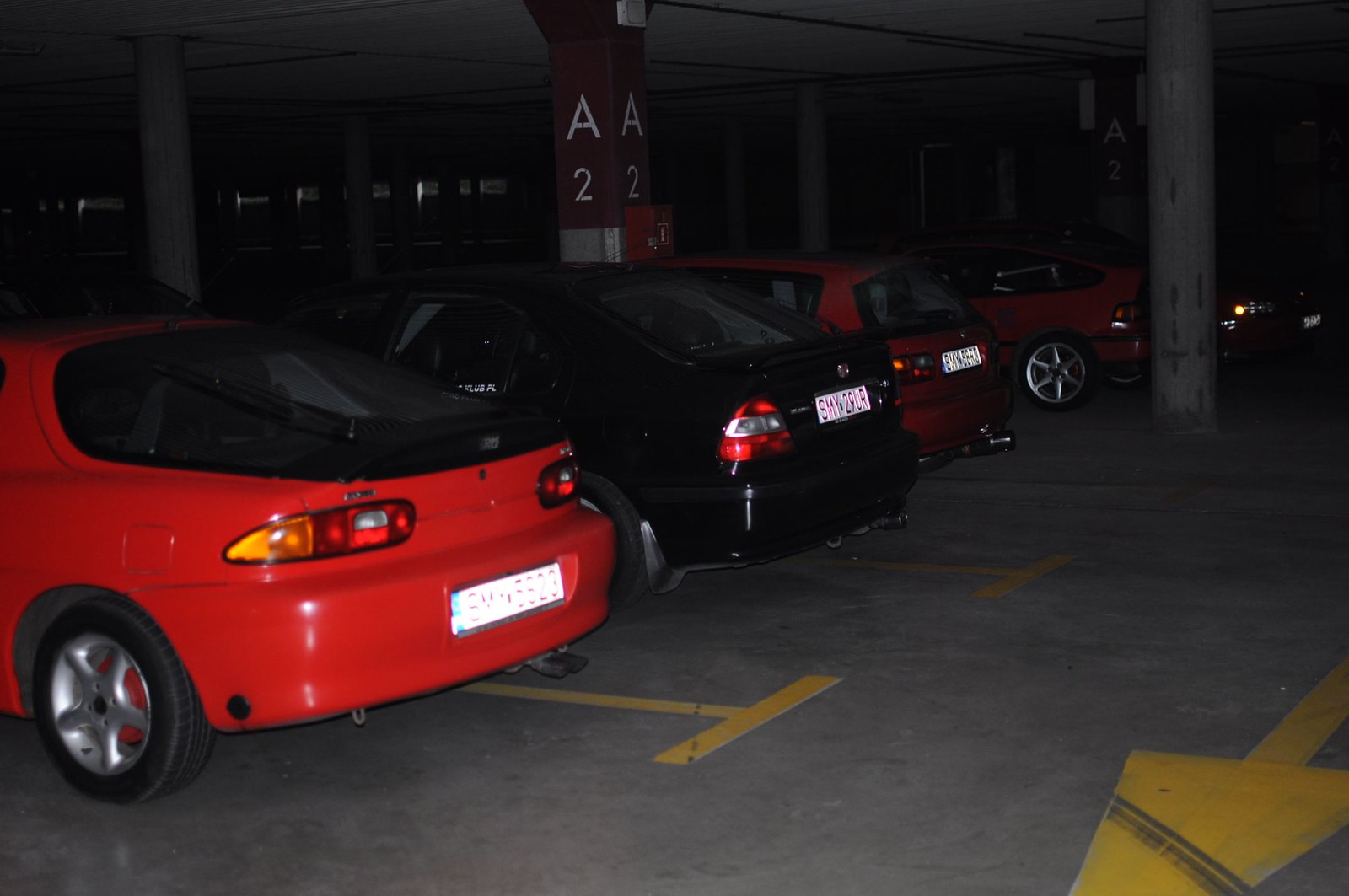This is a photograph of an underground parking garage characterized by its broad, spacious setting, and gray concrete floor marked with yellow parking spaces and directional arrows. The parking garage has a very dark ambiance, with minimal lighting that seems to originate only from the camera's flash. In the foreground, four cars are prominently visible. On the far left, there is a bright red, shiny car resembling a Camaro, followed by a black car with distinctive red taillights. Adjacent to the black car is another red vehicle, with a final red car appearing further in the distance, noticeable for its black wheel with a silver interior.

The cars, which all show their back ends with visible taillights and elongated license plates that suggest they might be from Britain or Canada, are smaller, compact models. The garage also features significant structural elements, including a large cement pole on the right in the distance. Notable markings on the pillars include the letters "AA" with the numbers "22" and another with the letter "A" and the number "2," indicating specific rows of parking. The entire atmosphere is enhanced by the yellow lines and arrows on the cement floor, guiding the parking arrangement and traffic flow within the garage.